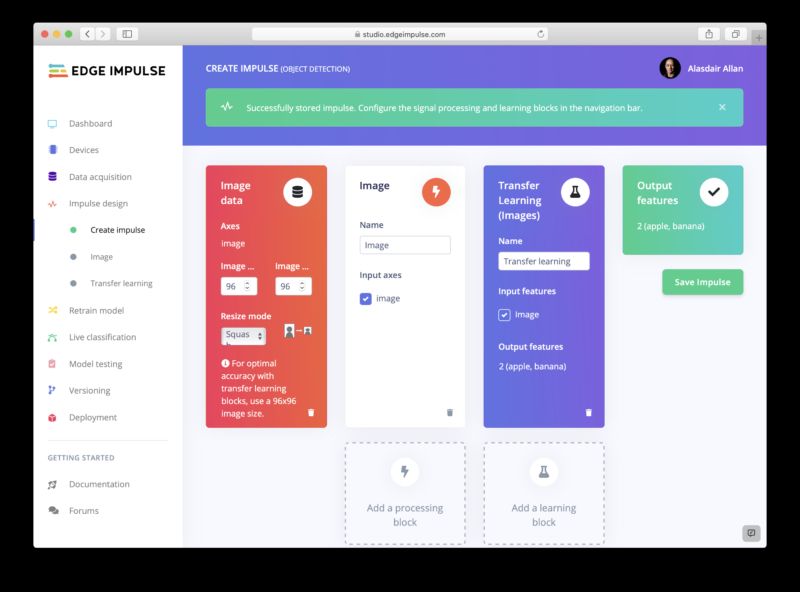Screenshot from the Edge Impulse website: The top left corner prominently displays the Edge Impulse logo in black font, accompanied by a small graphic. The interface appears to be accessed via a MacBook or Safari browser. Below the logo, an extensive navigation menu is visible, featuring clickable options in the following order: Dashboard, Devices, Data Acquisition, Impulse Design, Create Impulse, Image Transfer Learning, Reach, Train, Model, Live Classification, Model Testing, Versioning, Deployment, Getting Started, Documentation, and Forums.

To the right of the navigation menu, a section labeled "Create Impulse" is situated near the assumed user profile area. Below this, additional sections titled "Image Data," "Image," "Transfer Learning Images," and "Output Features" are displayed, each highlighted in different colors: red, white, blue, and green, respectively.